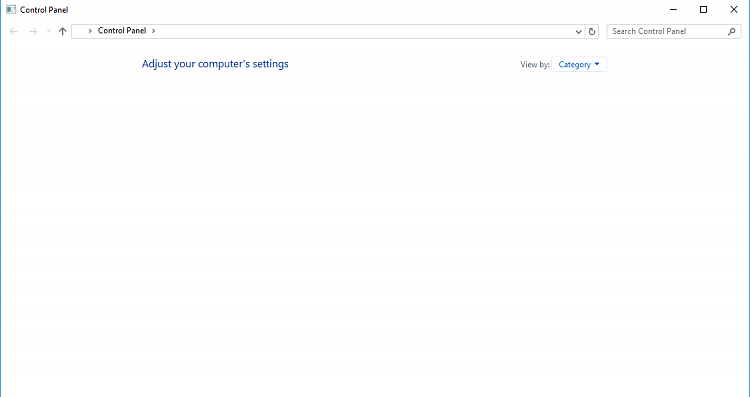This screenshot captures the minimalistic design of a settings or control panel webpage. The background is predominantly white, occupying roughly 98.9% of the screen. In the upper left corner sits a small gray page icon, adjacent to which, in black font, is the text "Control Panel." On the upper right, there are three black icons: a subtraction icon, a square icon, and an 'X' icon.

Beneath the "Control Panel" label in the upper left, you will find a set of navigational icons: a backward arrow, a forward arrow, and a refresh arrow. To their right, a rectangular box contains the text "Control Panel" in black font, and at the right end of this box is a small black downward arrow. Adjacent to this box is a square icon with a refresh symbol.

Further to the right, another square box contains the text "Search Control Panel," ending with a magnifying glass icon on its right side.

The lower part of the screenshot reveals a large empty white area, with the words "Adjust Your Computer Settings" prominently displayed in blue font. This area appears to be intended for displaying the user's customizable settings options.